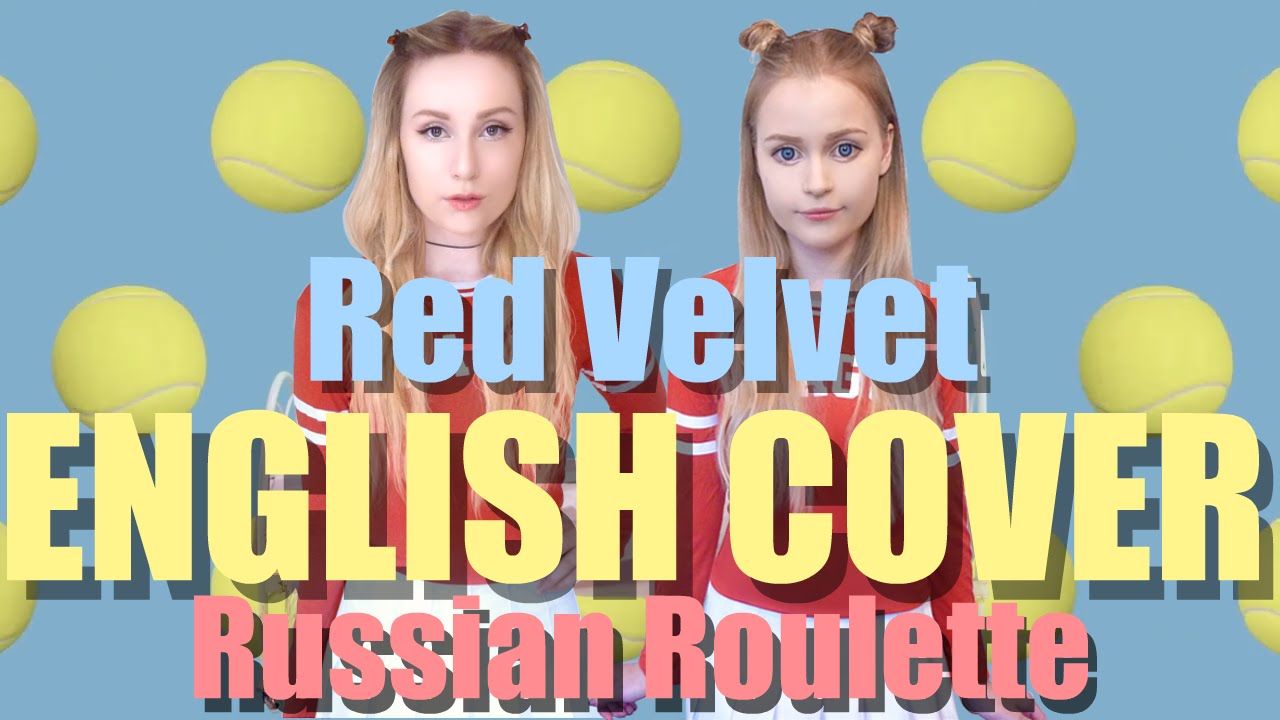The image depicts a digitally enhanced, full-color, horizontally rectangular photograph that appears to serve as an album cover. The background of the image transitions from a darker blue at the top to a lighter blue at the bottom and is adorned with a repeating pattern of yellow tennis balls, each about the size of the girls' heads. Dominating the center are two young blonde-haired Caucasian females with long hair, standing side by side in red tops and white bottoms, resembling cheerleading uniforms. Notably, the girl on the right has exceptionally large and wide-open eyes, while the girl on the left has a more relaxed expression with half-closed eyes and a choker necklace. Both have closed mouths and are not smiling. The text on the image reads "red velvet" in blue at the top, "English cover" in yellow just below, and "Russian roulette" in pink at the bottom.